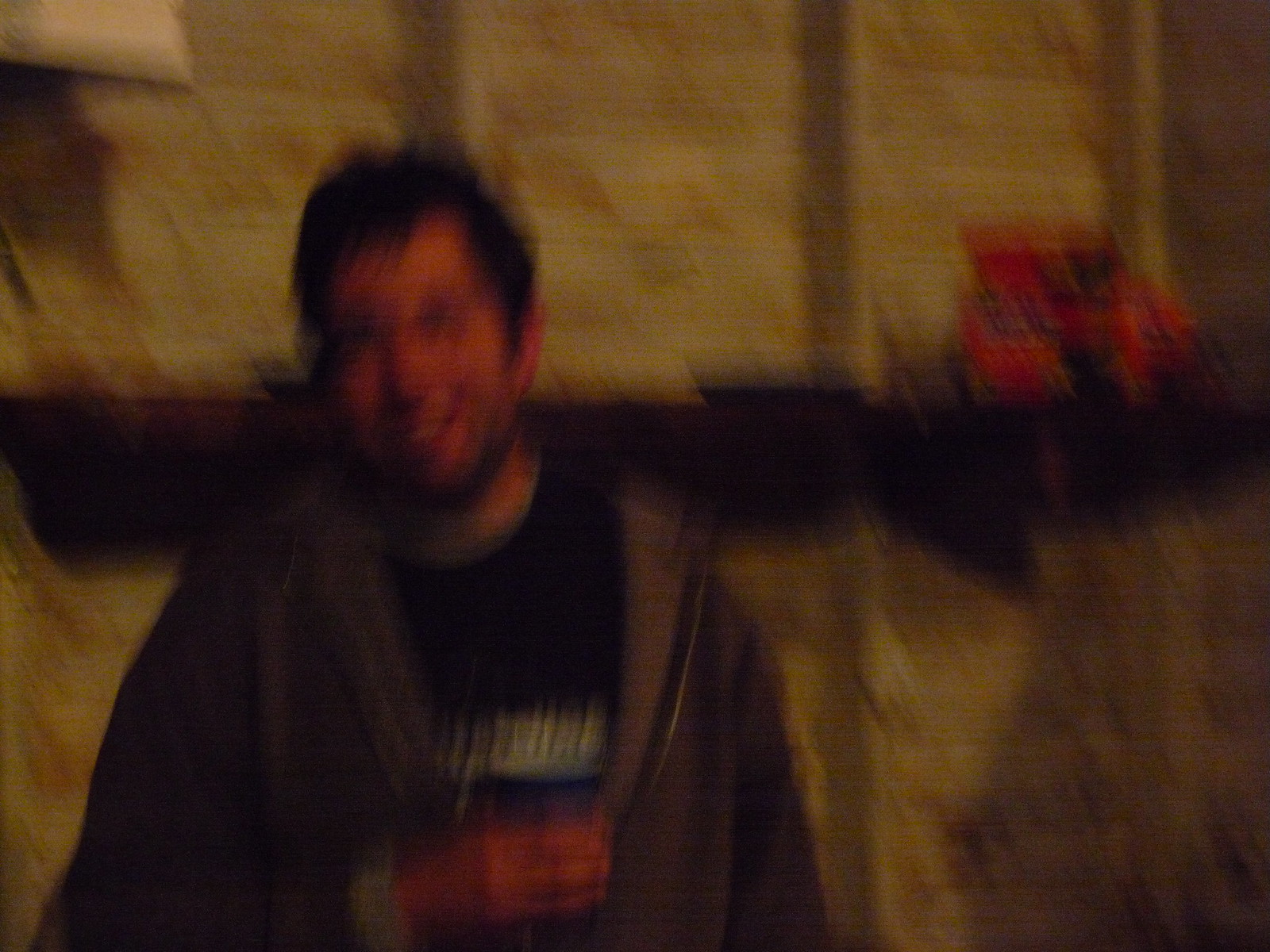This image is a blurry photograph of a Caucasian man standing in what appears to be an unfinished room—possibly a basement or garage—as evidenced by the exposed wooden framing on the off-white, light brown walls. The man is situated slightly to the left of the center, seen from the waist up. He has short, dark brown hair and a tightly cropped beard, with an indistinct suggestion of small, gold-rimmed round eyeglasses due to the blur. He is dressed in a gray zip-up hooded sweatshirt over a black t-shirt featuring some white and red lettering, though the exact text is indiscernible. His right hand is extended in front of him, holding a blue cup. Behind him on the right, there is a dark-colored shelf with a distinct red object on it. The shelf stands out against the wooden beams and panels of the background, contributing to the unfinished appearance of the setting. Despite the blurriness, he appears to be smiling, and the overall impression suggests a casual, candid moment.